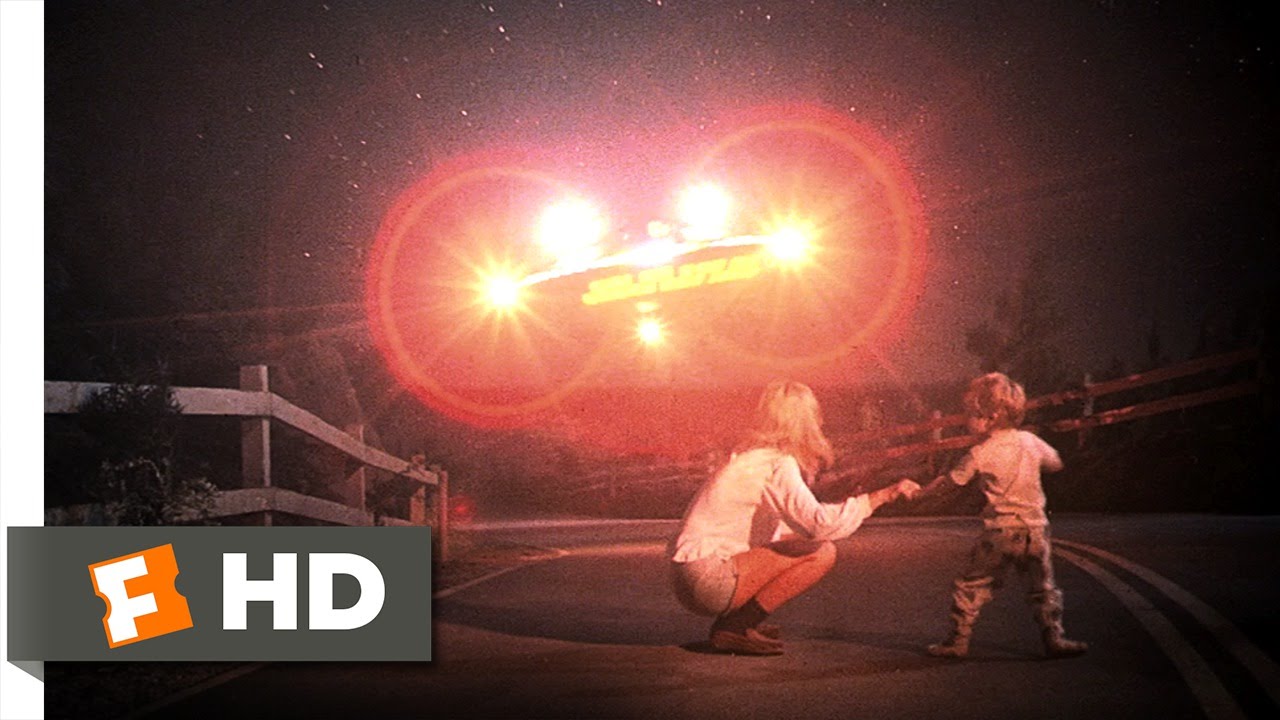This promotional photo for the movie "Close Encounters of the Third Kind," features a dramatic nighttime scene under a star-studded sky. Dominating the background is a large spaceship, emanating bright lights with a captivating lens flare of orange and yellow hues. In the foreground, a woman in short jean shorts, a white blouse, brown loafers, and black socks kneels on a rural highway, gripping the hand of a small boy dressed in a white t-shirt and colorful pajama pants, barefoot. Both appear awe-struck, the woman gazing at the spacecraft, while the boy looks at her. The road they stand on is flanked by wooden fence posts, resembling an old-school bridge. A double yellow line runs just right of the boy, signaling the middle of the road. A faint car can be seen in the distance. In the bottom left corner of the image, a gray rectangular badge bears the Fandango logo—a small orange ticket with an "F"—and the label "HD" in white letters, emphasizing its cinematic quality.